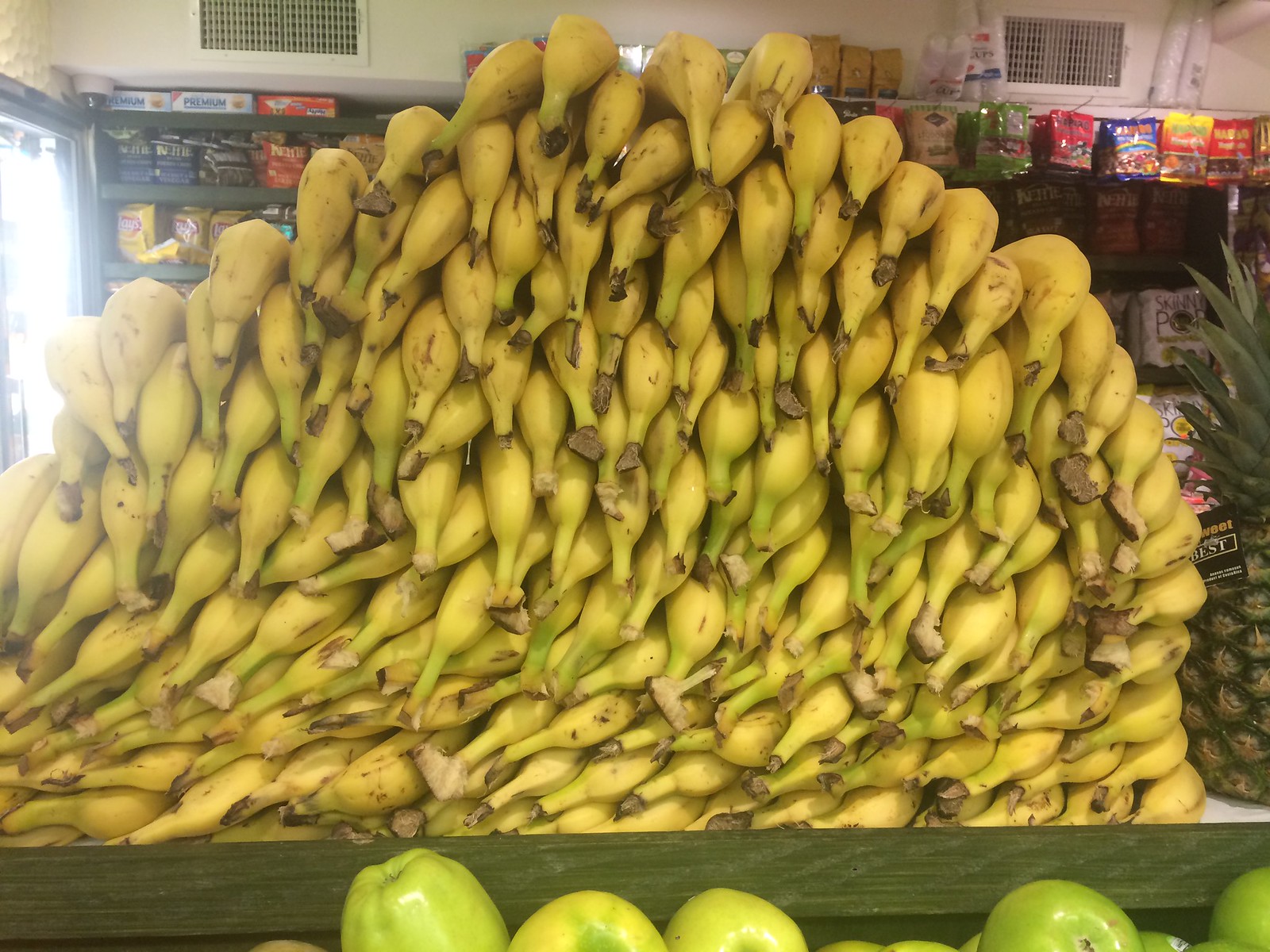This detailed photograph was taken in what appears to be a convenience store or small grocery store, focusing on an enormous, pyramid-like pile of bananas stacked on a wooden table with a greenish border. The bananas, predominantly yellow with some green and brown spots, are piled high, reaching approximately four to five feet. The sheer volume is striking, with an estimated 200 bananas occupying the center of the image. Behind this mountainous assembly of bananas, store shelves are stocked with various snacks, including Haribo gummy bears, Skinny Pop popcorn, kettle chips, Lay's chips, and Nabisco premium saltine crackers. To the right of the banana pile, there is a partially visible pineapple, and at the bottom, a few Granny Smith green apples are scattered. The photo is well-lit with natural light, hinting at daytime, and no text is present in the image.